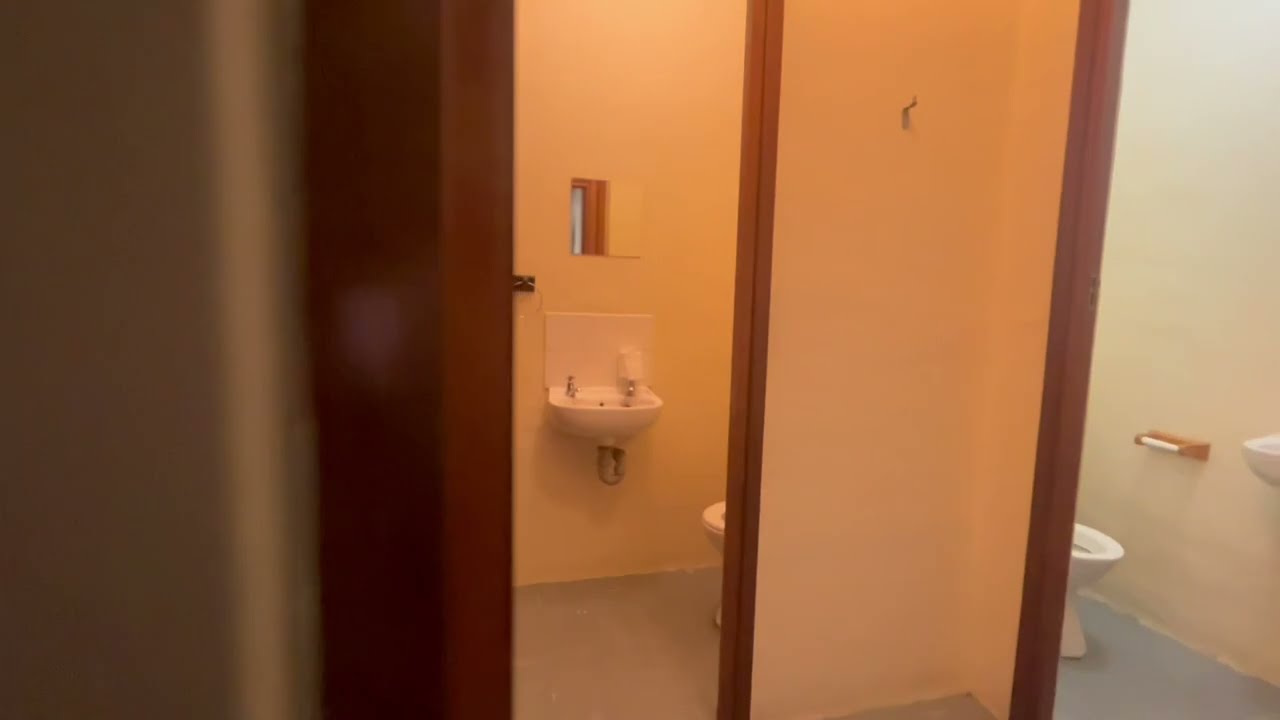The image shows a sparsely furnished, likely public bathroom that includes two separate stalls divided by a partial wall or divider. The stall to the right has a white wall and a light blue floor, featuring an exposed porcelain sink fixed to the wall, a toilet partially visible in the bottom right corner, and an empty toilet paper holder fixed to the wall. A small coat hook hangs on the divider wall. In the stall on the left, the setting appears more distinct: it has yellow walls with wooden trim and a gray floor. This area also includes a wall-mounted sink and a partially visible toilet, just in front of which sits a small window. The image mostly captures the sparse, functional interior typical of public restrooms, further accented by the absence of any human presence, hinting that the photo might be for planning a remodel or redesign.